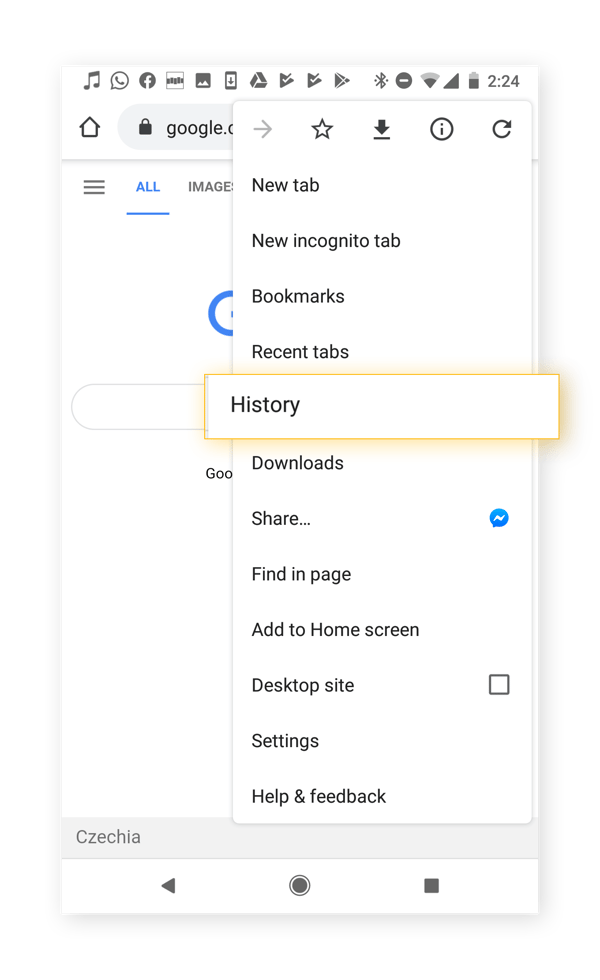This vertical screenshot captures the detailed interface of someone's smartphone screen. Evident from the multitude of notifications at the top, this person has alerts from WhatsApp, Facebook, music apps, downloads, Google Drive, app installations, and Google Play. The status icons show active Bluetooth, Do Not Disturb mode, connected Wi-Fi, strong mobile reception, and a battery level at approximately 60%. The current time displayed is 2:24, though it’s unclear whether it is a.m. or p.m.

The background of the screen is white, indicating a clean and minimalist design. The user is browsing on the Google Chrome app, positioned on the Google.com homepage. An options tab is open, prominently displaying various browser functionalities. The 'History' option is highlighted with a yellowish outline and glow, suggesting it is currently selected. Below, 'Czechia' (C-Z-E-C-H-I-A) is noted on the bottom left-hand corner. The phone's navigation buttons are visible at the bottom, in gray. While the majority of the text and buttons are rendered in black or gray, the 'All' button on Google stands out in blue with a matching underline, signifying its active status.